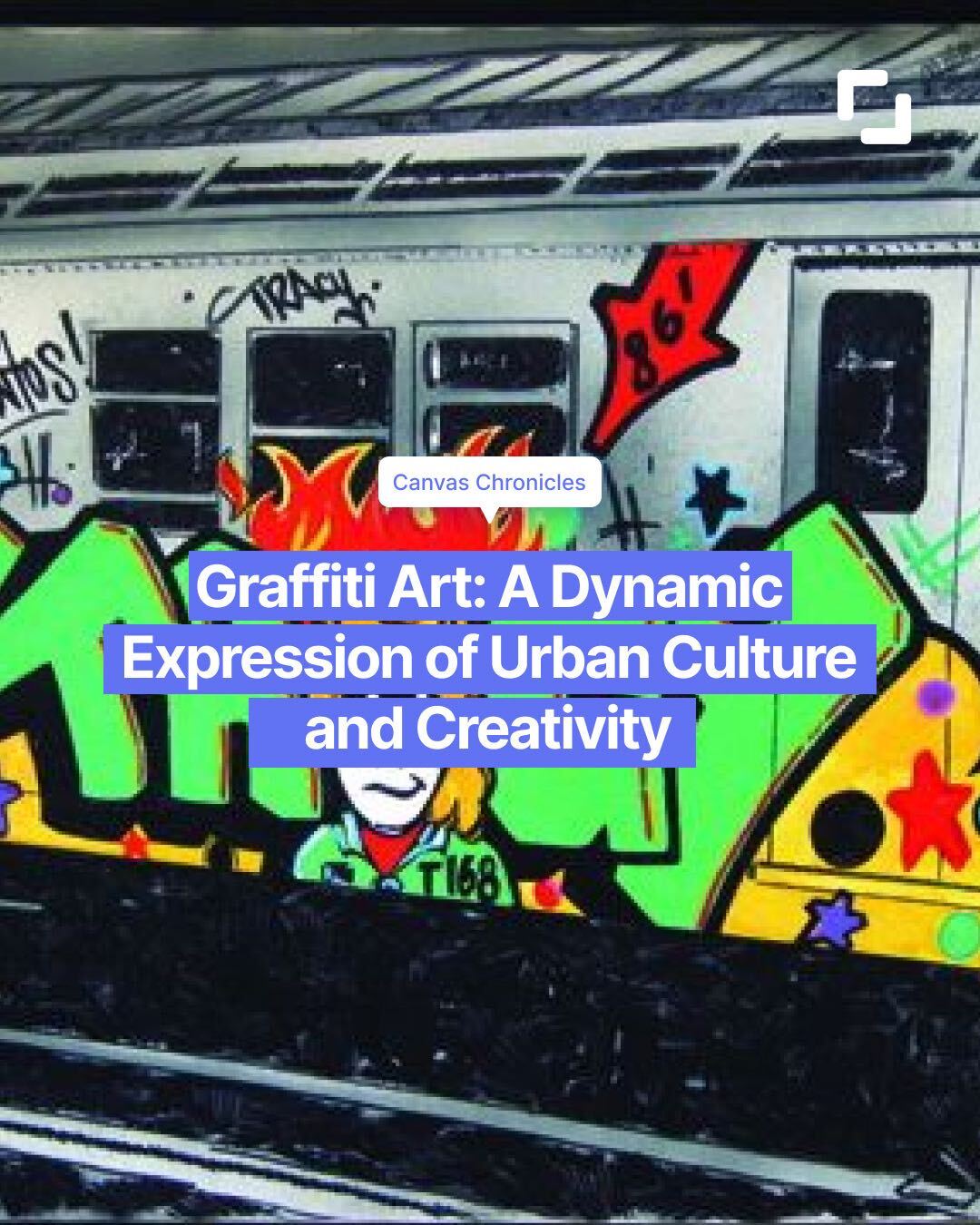The image is an advertisement featuring a heavily graffitied subway car, surrounded by elements that enhance its urban atmosphere. The subway car, partially obscured by text and banners, showcases a myriad of vibrant graffiti art, predominantly in neon colors like green, red, and orange-yellow. Among the graffiti, the most prominent piece is a striking green tag that spells out "Tracy," accompanied by a detailed illustration of a girl with yellow hair, wearing a green sweatshirt over a white t-shirt. Additional graffiti includes a red arrow pointing towards a flame with the number "861" inscribed in it.

Overlaying the image, there are three long horizontal blue banners placed just below the windows of the subway car, with the white text reading “Graffiti Art, a dynamic expression of urban culture and creativity.” Above this caption, in a word bubble, the title "Canvas Chronicles" is emblazoned, hinting at either the name of a magazine or the thematic centerpiece of the advertisement. An overhang, likely part of the subway platform, is visible above the train, adding perspective to the scene. In the top right corner, a distinctive logo resembling a box with cutouts in the top right and bottom left corners is present. The background subtly fades to black towards the bottom, revealing a glimpse of the tracks, grounding the scene in an authentic urban setting.